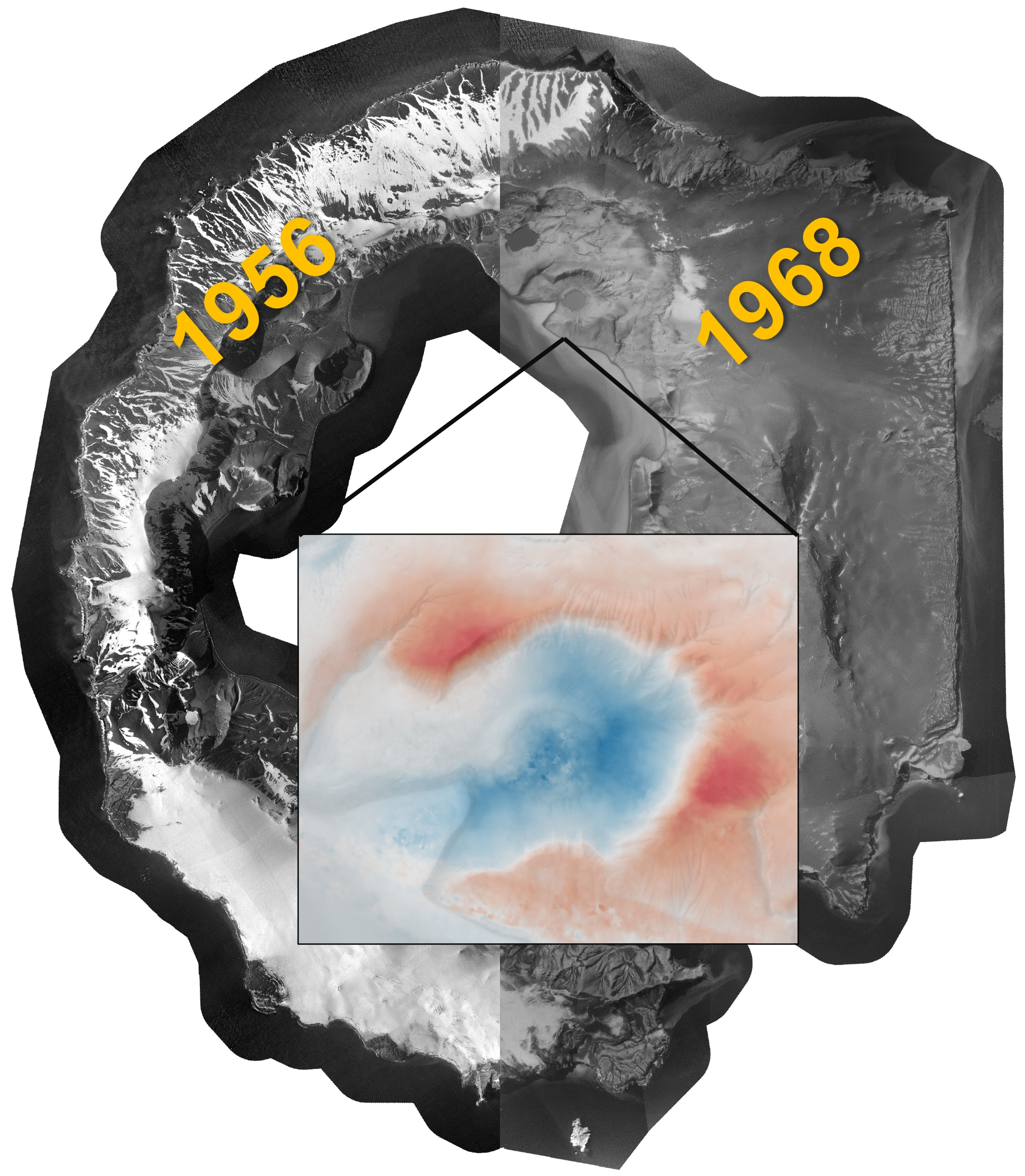The image depicts a unique stone sculpture that appears to be a jagged cross-section of rock, with a distinct hole in its center. The sculpture is mostly dark charcoal black with white streaks running through parts of it. Emblazoned in light orange or gold are the years "1956" on the white streak and "1968" on a part without the streak. Extending from just above the center are two black lines that form two sides of a square and serve as a hanger for a watercolor painting. The painting, resembling the shape of the stone, is predominantly light blue in the middle where the hole is, transitioning to pink and red hues around the edges. The entire composition is set against a bright, clean, white background, which enhances the clarity and detail of the piece.